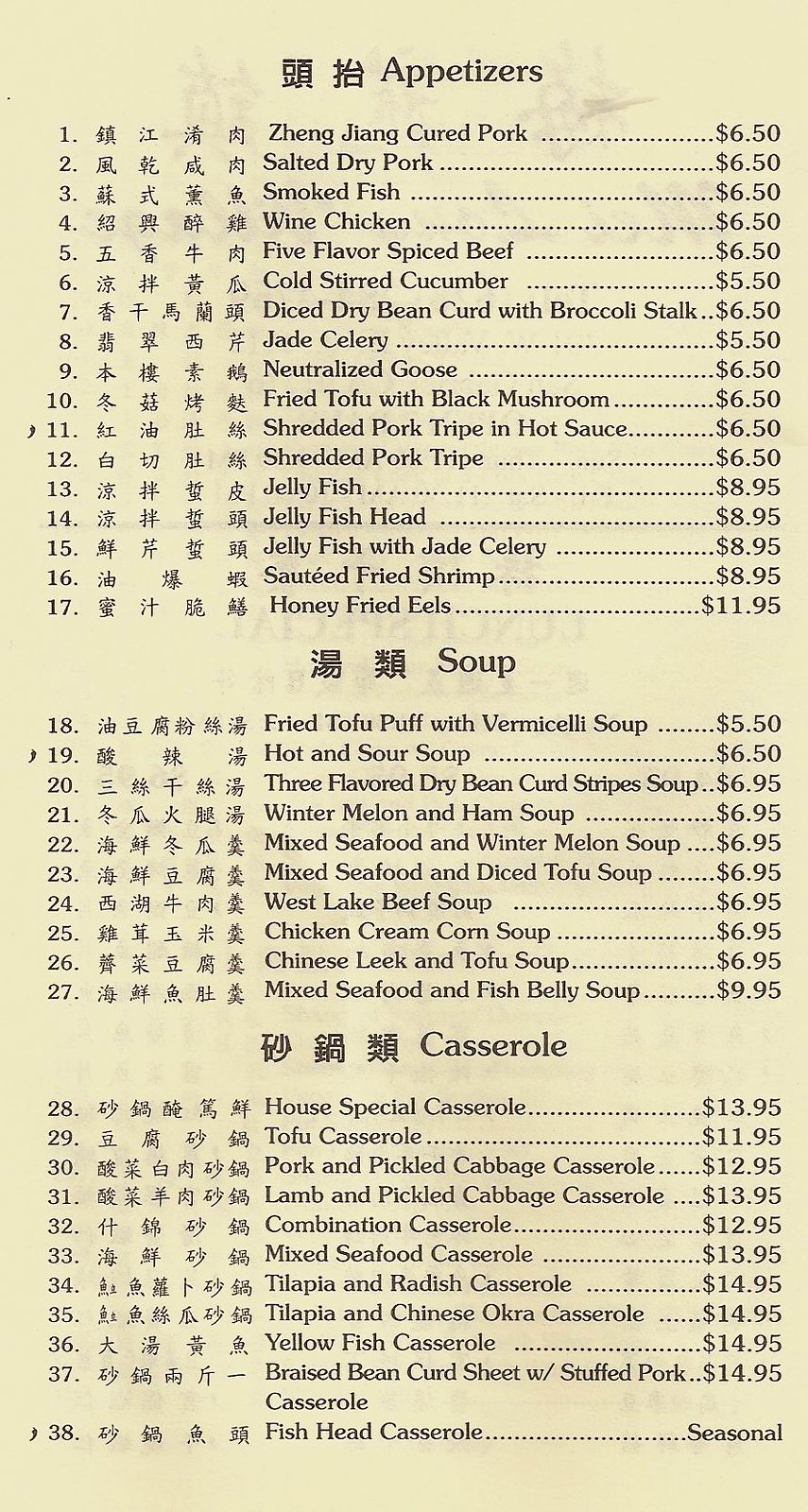This detailed image captures a scanned page of a menu from a Chinese restaurant, presenting an array of dishes in both Chinese and English. The menu is organized into sections that begin with appetizers, followed by soups, and then casseroles. Each menu item is paired with its name in Chinese characters on the left side.

**Appetizers (Items 1 to 14):**
1. Zhangjiang Cured Pork - $6.50
2. Salted Dry Pork - $6.50
3. Smoked Fish - $6.50
4. Wine Chicken - $6.50
5. Five Flavor Spiced Beef - $6.50
6. Cold Stirred Cucumber - $5.50
7. Diced Dry Bean Curd with Broccoli Stalk - $6.50
8. Jade Celery - $5.50
9. Neutralized Goose - $6.50
10. Fried Tofu with Black Mushroom - $6.50
11. Shredded Pork Tripe in Hot Sauce - $6.50
12. Shredded Pork Tripe - $6.50
13. Jellyfish - $8.95
14. Jellyfish Head - $8.95
15. Jellyfish with Jade Celery - $8.95
16. Sauteed Fried Shrimp - $8.95
17. Honey Fried Eels - $11.95

**Soups (Items 18 to 27):**
18. Fried Tofu Puff with Vermicelli Soup - $5.50
19. Hot and Sour Soup - $6.50
20. Three Flavor Dried Bean Curd Stripe Soup - $6.95
21. Winter Melon and Ham Soup - $6.95
22. Mixed Seafood with Winter Melon Soup - $6.95
23. Mixed Seafood with Diced Tofu Soup - $6.95
24. Westlake Beef Soup - $6.95
25. Chicken Cream Corn Soup - $6.95
26. Chinese Leek and Tofu Soup - $6.95
27. Mixed Seafood and Fish Belly Soup - $9.95

**Casseroles (Items 28 to 38):**
28. House Special Casserole - $13.95
29. Tofu Casserole - $11.95
30. Pork and Pickled Cabbage Casserole - $12.95
31. Lamb and Pickled Cabbage Casserole - $13.95
32. Combination Casserole - $12.95
33. Mixed Seafood Casserole - $13.95
34. Tilapia and Radish Casserole - $14.95
35. Tilapia and Chinese Okra Casserole - $14.95
36. Yellowfish Casserole - $14.95
37. Braised Bean Curd Sheet with Stuffed Pork Casserole - $14.95
38. Fish Head Casserole (Seasonal Pricing)

This page offers a mouth-watering glimpse into the diverse options available, showcasing traditional Chinese culinary delights for a range of tastes and preferences.